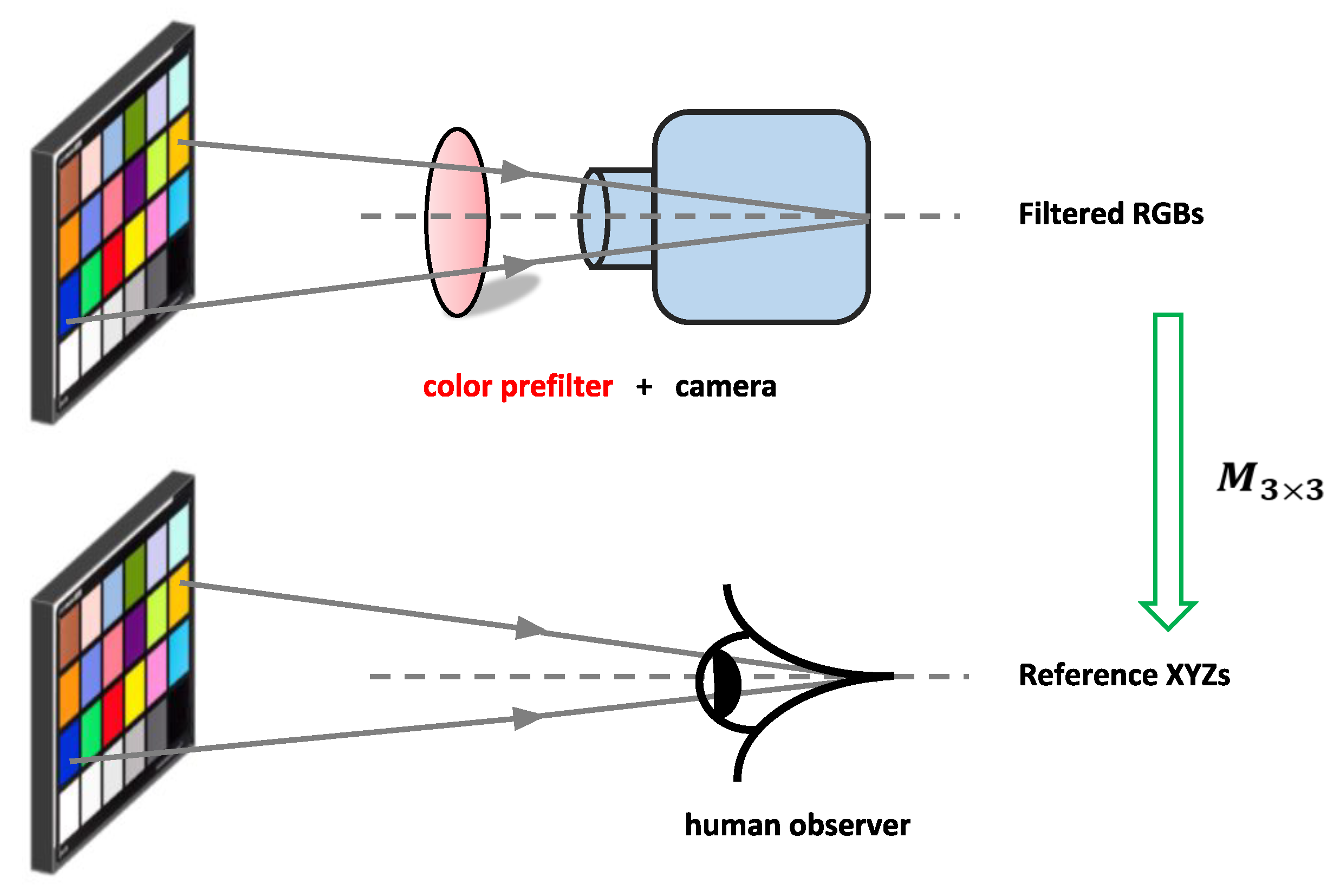The image is a detailed schematic diagram illustrating the process by which a camera with a color pre-filter and a human eye observe and interpret colors. Set against a white background, the diagram features two main sections: the upper portion depicts a camera system while the lower portion represents the human eye. Starting at the top, the camera setup includes a vertical red oval labeled "Color Pre-Filter" followed by a blue square labeled "Camera." To the right of this setup, the filter's effect is captured as "Filtered RGBs" with an arrow pointing downwards labeled "Reference XYZs." Additionally, there's a 3x3 matrix symbol (M 3x3) connected to the arrow, indicating color space transformation. Below this, a similar mechanism is depicted for a human observer. This section includes a detailed illustration: the side view of a human eye looking at a 3D color palette. The palette features a four-row grid of various colors like brown, blue, green, and pink. The pathway from the eye to this grid is marked with a dotted line culminating in a green arrow labeled "Reference XYZs." This diagram meticulously demonstrates how a camera's filter system is designed to mimic the human perception of light and color.